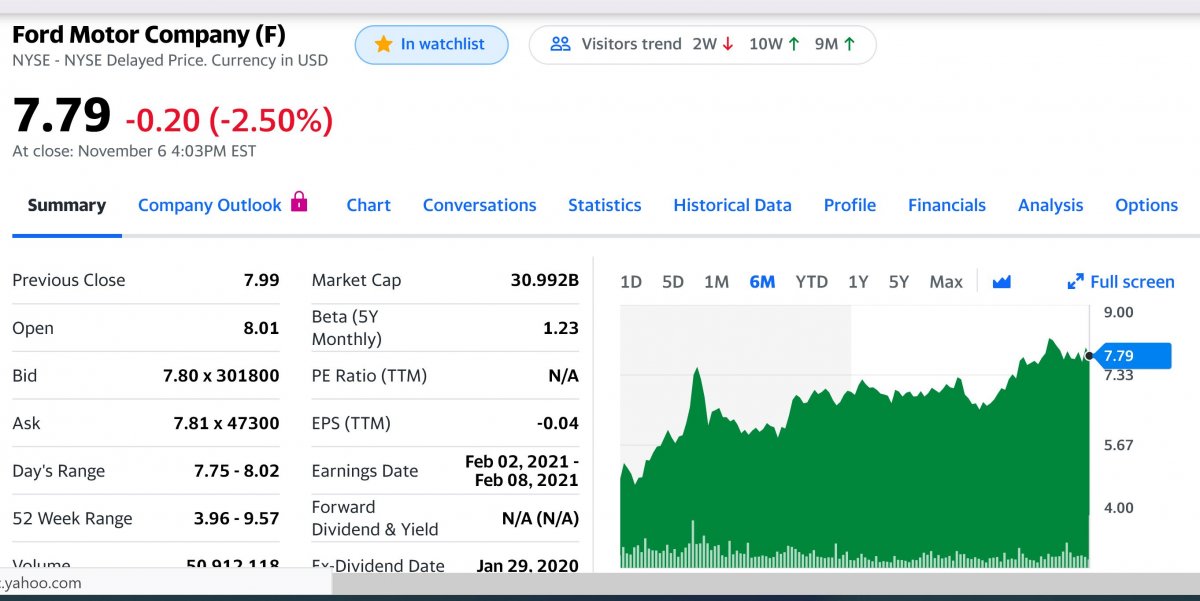**Detailed Descriptive Caption:**

The webpage displays detailed financial information about Ford Motor Company, traded under the ticker symbol 'F' on the New York Stock Exchange (NYSE). The data is presented in US dollars with a slight delay. At the top, there is an option to add the stock to a watchlist and observe visitor trends, characterized by a declining pattern over two weeks, a rising trend over ten weeks, and an upward movement over nine months.

Prominently displayed is the stock's closing price of $7.79, which reflects a decrease of $0.20, or 2.50%, as of the close on November 6 at 4:03 PM Eastern Time.

The webpage is organized into multiple tabs: Summary (currently selected), Company Outlook, Chart, Conversions, Statistics, Historical Data, Profile, Financials, Analysis, and Options.

Under the Summary tab, the following stock data is displayed in a two-column layout:

- **Previous Close:** $7.99
- **Open:** $8.01
- **Bid:** $7.80 × 301,800 shares
- **Ask:** $7.81 × 47,300 shares
- **Day’s Range:** $7.75 - $8.02
- **52-Week Range:** $3.96 - $9.57
- **Volume:** (Partially Cut Off)
  
On the right column:
- **Market Cap:** $30.992 Billion
- **Beta (5Y Monthly):** 1.23
- **PE Ratio (TTM):** N/A
- **EPS (TTM):** -$0.04
- **Earnings Date:** February 2, 2021 – February 8, 2021
- **Forward Dividend & Yield:** N/A
- **Ex-Dividend Date:** January 29, 2020

A detailed graph appears beneath this data, capable of showing stock performance across a range from one day to the maximum historical data available. The 6-month (6M) view is currently highlighted, with the graph displaying performance fluctuations represented in green.